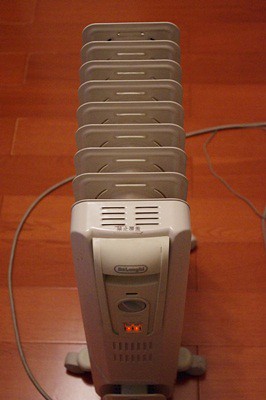This photograph captures a single space heater positioned on a shiny, medium-dark brown wooden floor. The space heater, which resembles an old-fashioned radiator, is predominantly off-white or light gray in color and has a rectangular shape. The device stands on a small rolling base with wheels, making it portable.

In the middle of the image, the most prominent space heater shows an illuminated red light, likely indicating that it is turned on. The front panel, although a bit blurry, features a visible but unreadable brand name at the top within an oval shape, followed by a round dial to adjust the temperature. Below the dial, there is a lit area, which perhaps functions as an operational indicator.

The space heater has several slats, or openings, between which heat can emanate, and there appears to be a series of these slats extending into the background, creating an illusion of multiple units, although it is, in fact, a single piece viewed from a specific angle. A long cord snakes out from the bottom left corner of the image, stretching toward the middle-right, but its endpoint is cropped out of the photo.

Overall, this image emphasizes the functional and design aspects of the space heater, with a notable contrast between the shiny wooden floor and the appliance's off-white/light gray color.